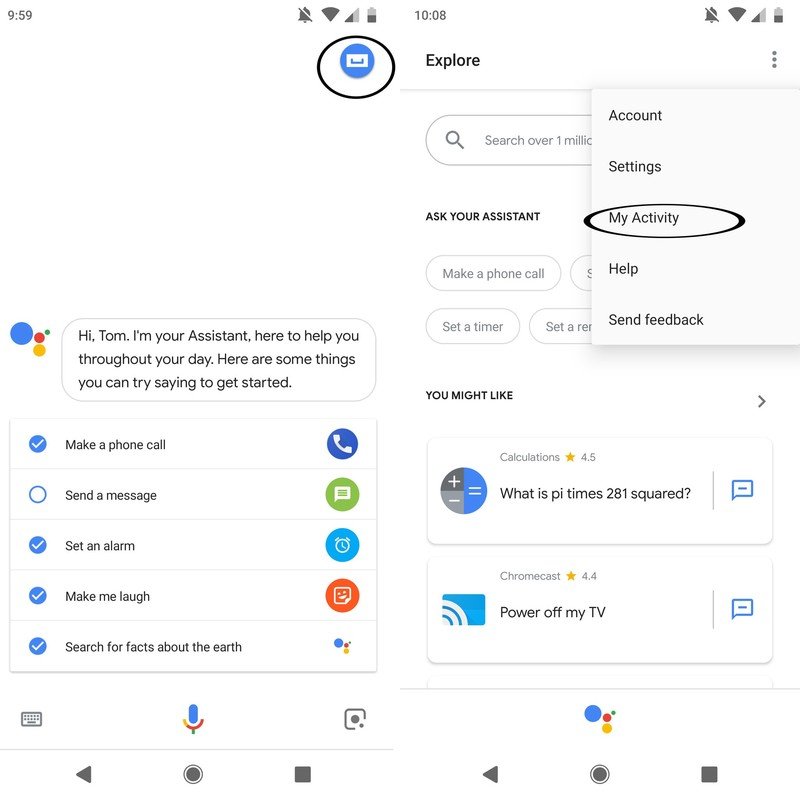This image is a compilation of two side-by-side mobile device screenshots showcasing a Google application from different viewpoints. Above the app interface, both screenshots consistently display icons for time, Wi-Fi connection, network signal, and battery status, albeit with different times: the first screenshot is captured at 9:59 and the second at 10:08.

In the first screenshot, the app's interface features a dialogue bubble that greets the user with, "Hi Tom, I'm your assistant here to help you throughout your day. Here are some things you can try saying to get started." Below this greeting, various actionable commands such as "Make a phone call," "Send a message," "Set an alarm," "Make me laugh," and "Search for facts about the Earth" are listed to assist the user in utilizing the assistant effectively. A microphone icon button is also visible, allowing the user to activate the assistant via voice command.

The second screenshot unveils a dropdown menu with options including "Account," "Settings," "My Activity," "Help," and "Send Feedback." Notably, the "My Activity" option is circled in black ink, drawing attention to it. This screenshot also presents an extended list of additional tasks that the assistant can perform for the user.